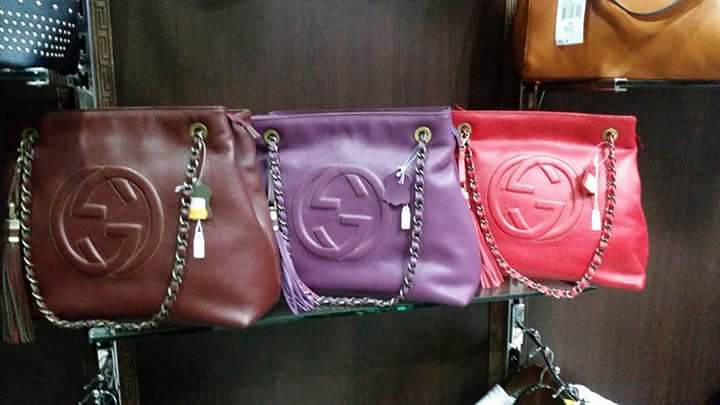The image captures a refined sales display in a retail store featuring purses against a sleek, dark brown wood panel backdrop with visible, polished grain patterns. The main focus is a glass shelf supported by two silver metal bars, prominently showcasing three stylish Gucci leather purses, each adorned with silver chains. 

- The leftmost purse is brown, slightly tilted to the left, displaying the iconic Gucci emblem with a chain hanging down and a yellow price tag.
  
- In the center, a purple Gucci purse features the emblem prominently with a matching purple tassel hanging from the silver chain.

- The rightmost purse is red, also featuring the Gucci emblem and a silver chain with a red tassel.

Additionally, partially visible in the upper left is a black purse decorated with silver diamonds and dots, and in the upper right, a dark beige-brown purse with a price tag hanging down, showcasing just part of the strap. The meticulously arranged display emphasizes the luxury and elegance of the Gucci brand.